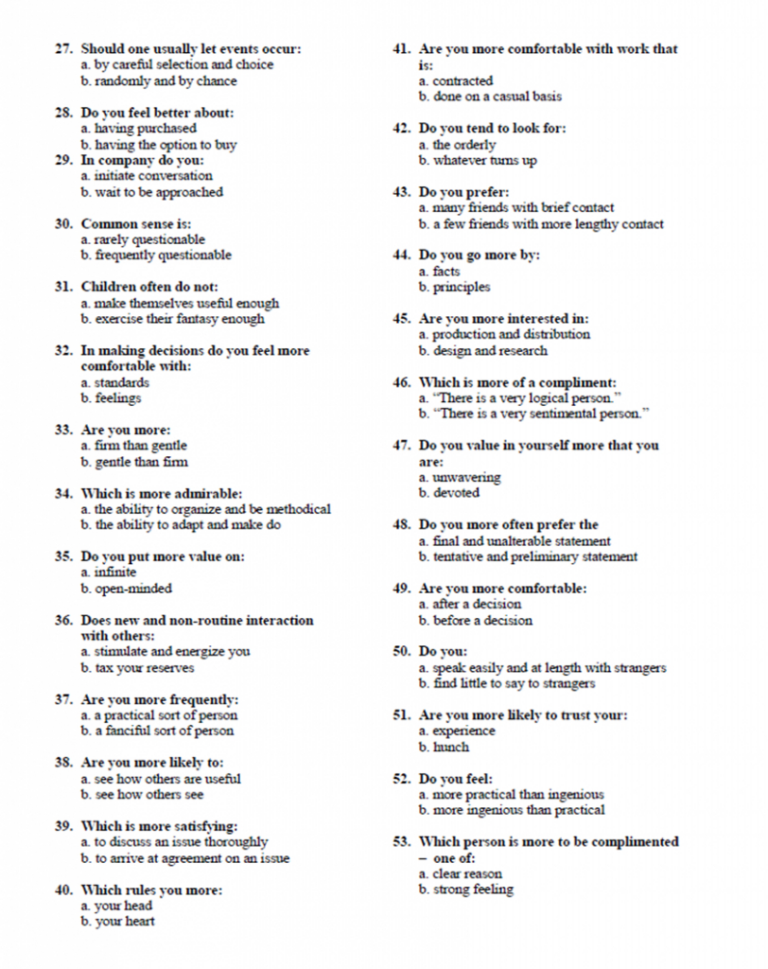This image is a screenshot of a segment from an unidentified web page displaying a portion of a test or questionnaire. The background is white, and the layout features two columns filled with questions. Each question is numbered sequentially from 27 to 53. Each question has two multiple-choice answers labeled A and B, both options written in lowercase letters followed by a period. The text is presented in a dark gray font that appears somewhat faded and small, impacting overall readability. 

At the top left corner, question number 27 reads, "Should one usually let events occur:" with answer choices "a. by casual selection and choice" and "b. randomly and by chance" listed neatly beneath the question. The structured format remains consistent throughout, with each new question following the same layout pattern. The series concludes in the lower right-hand corner with question number 53, which asks, "Which person is more to be complimented?" with the answers provided as "a. clear reason" and "b. strong feeling." The lack of headers or footers and the visible wear on the text suggest that this might be a screenshot of an older or lower-quality document.